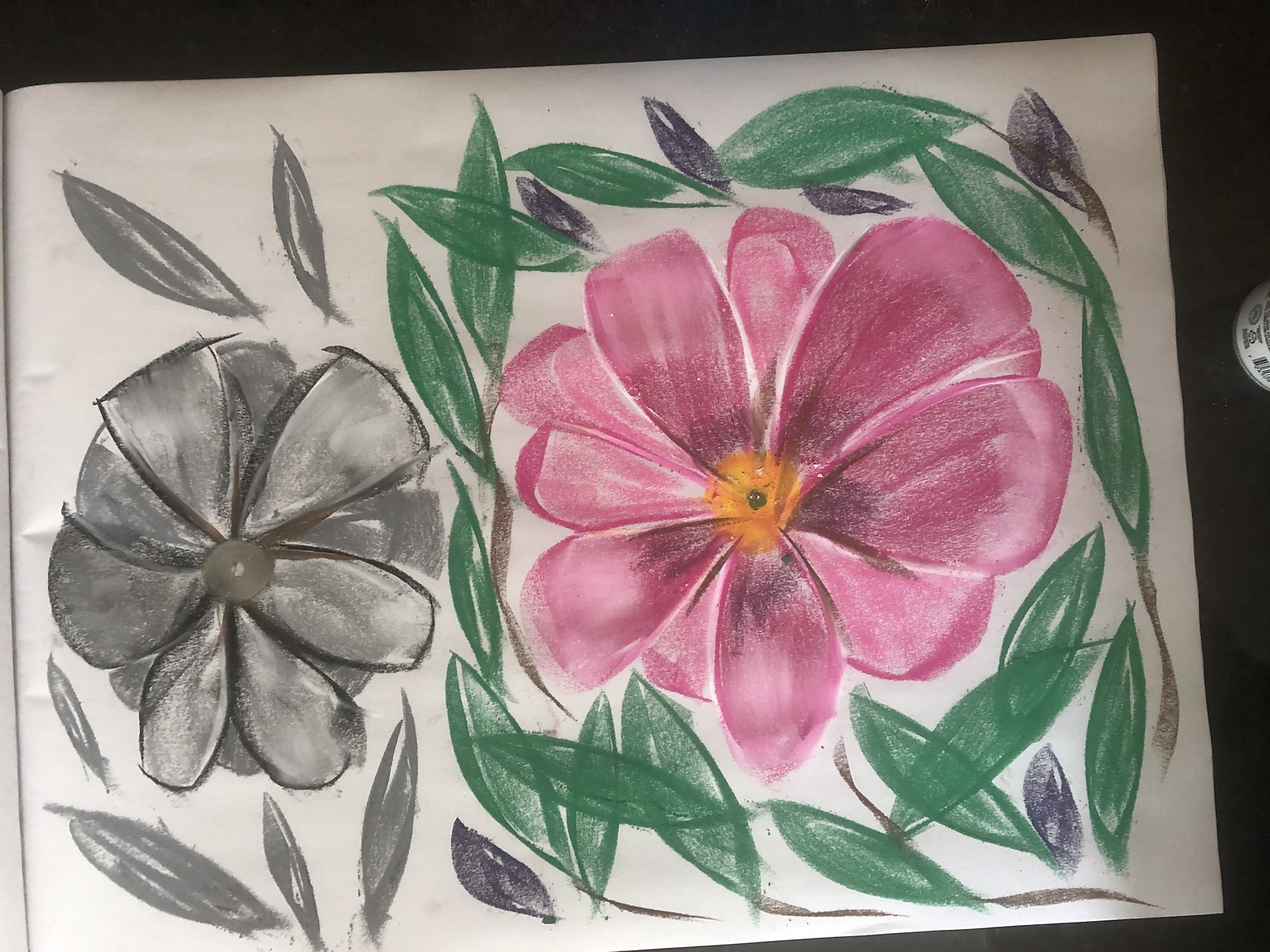The sketch on this white sheet of paper features two distinct flowers rendered in a mix of gray, black, green, pink, and yellow-orange colors. The first flower stands out with its large pink petals, which have a subtle dusting of black near the edges, adding depth and texture. At the center of this flower is a vibrant yellow-orange bulb. Surrounding the pink flower are green leaves, with a few tinged in a purplish hue, adding a dynamic contrast. The second flower is more subdued, depicted entirely in varying shades of gray. Its center is a solid gray bulb, surrounded by small, understated gray petals that radiate outwards. The overall composition blends these colors harmoniously, creating a beautifully balanced and detailed representation of flora.